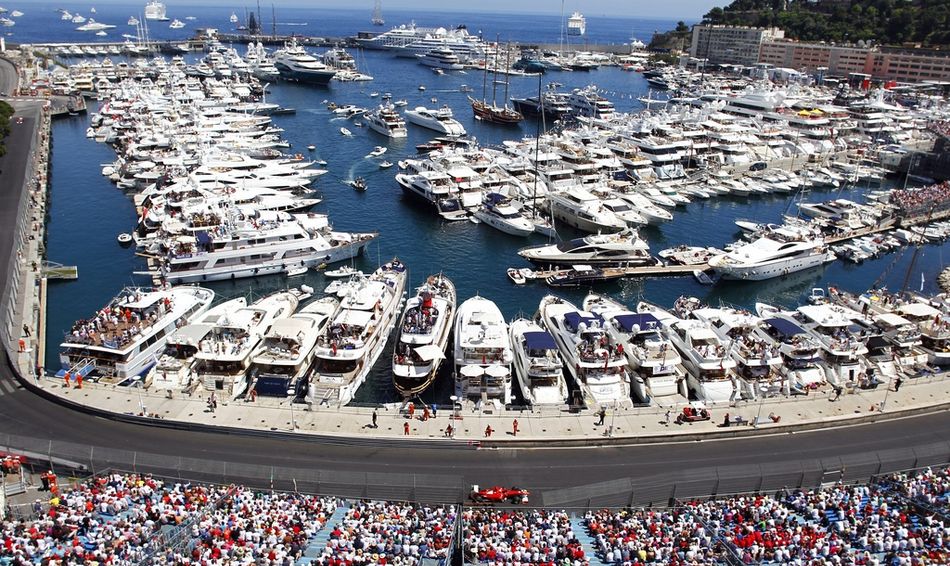The image captures an exhilarating Formula One race taking place at the edge of a bustling harbor. Most prominently, there's a U-shaped racetrack hugging the harbor's contours, bustling with excitement. The track is a wide, gray road, accommodating the sleek, red Formula One car prominent near the bottom center of the image, racing along the outer lane. Another car is visible in the distance, at the top left of the U-shaped track, though it's much smaller.

To the bottom of the image, large stands brimming with spectators stretch along the track's edge, with hundreds—if not thousands—of eager fans filling every seat. A fence separates the crowd from the track, ensuring their safety as they enjoy a thrilling view of the race. Just beyond the track, there's a wide walkway lined with more people, adding to the vibrancy of the scene.

The harbor itself is a spectacular sight, teeming with a flotilla of white yachts and various other boats, many moored right along the shore. The waters of the harbor shimmer in a deep blue, and a few jet skis can be seen darting between the boats. Some boats even have people standing atop them, enjoying a unique vantage point of the race.

In the upper sections of the image, the visual narrative continues with large buildings dotting the upper right-hand corner, standing several stories tall against a backdrop of lush, green hills. The scene stretches out to showcase the vast, open sea beyond the harbor, where even more boats are visible on the horizon, illustrating the scale and grandeur of this maritime setting. The sky peeks through at the very top, completing this dynamic, detailed panorama of a waterfront transformed into a high-speed racing arena.